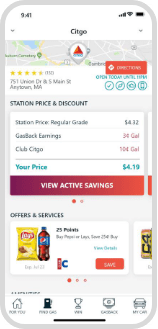Here is a cleaned up and detailed caption for the provided image description:

---

The image portrays a mobile screen depicted within a mock-up phone template, shown front-on against a white background. The mock-up phone features rounded corners and a simple gray border, encapsulating the phone UI. The image appears somewhat blurry, likely due to resizing, which has made the finer details challenging to discern.

At the top left corner of the screen, in dark blue text, the time reads "9:41." On the right side, icons indicating full signal strength, active Wi-Fi connection, and a fully charged battery are present. Below this status bar, centered on a white background, the text "CITGO" in blue letters is visible, flanked by drop-down arrows on both the left and right sides.

The main content of the display appears beneath, starting with a section depicting a map. At the map's center is a location icon embedded with the CITGO logo. Accompanying this are five yellow stars indicative of a rating, though the numerical rating itself is blurred. The address "751 Union Drive and S Main Street, Massachusetts" is listed nearby. Adjacent to this information is a red button with blue text, displaying "Open," likely indicating operational hours as "7 a.m. until 11 p.m." Small circular icons are also present within this segment, set against a white background.

A light gray background follows, highlighting bold blue capitalized text reading "STATION PRICE AND DISCOUNT." Below this header, a white rectangle contains several rows of data:

- The station price for regular grade gasoline is listed as $4.32.
- The cash gas back earnings are noted at $0.33 per gallon.
- Club CITGO offers a discount of $0.10 per gallon.
- The user's price is summarized as $4.19.

Beneath these details, a button with a gradient from dark maroon to light red reads "VIEW ACTIVE SAVINGS" in white capital letters. Below this, two dots signal the ability to switch between images, with the first dot highlighted.

The next section is titled "OFFERS AND SERVICES" in dark capital letters. Encased within a white rounded rectangle is an image of a bag of Lay's Original chips next to a Pepsi bottle. Partially visible text suggests savings information, with a prominent red button stating "SAVE ON" at the bottom right. Additionally, part of a product labeled "C4" is visible, though partially cut off.

At the screen's bottom, three menu buttons for navigating different offers and services are discernable. Finally, the application’s navigation menu includes icons for the home screen (a house), gas stations (a fuel pump), a trophy, cashback offers (a dollar symbol), and vehicle management (a car icon), though some text remains illegible due to the image blur.

---

This expanded caption provides a thorough, structured overview of the image, emphasizing clarity and detail.